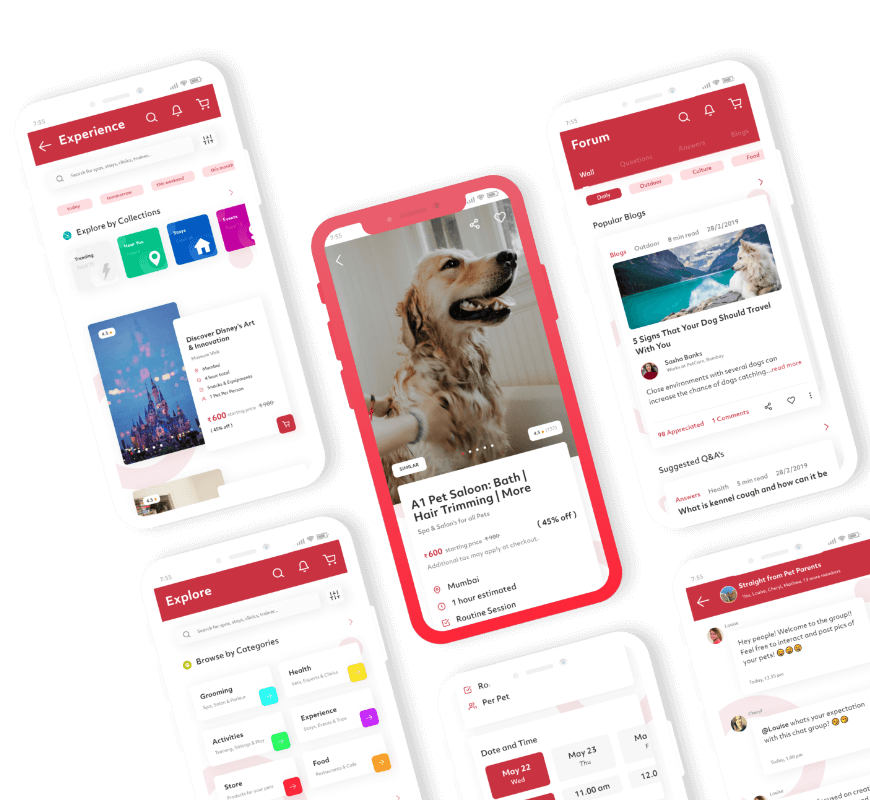The image appears to be a professional promotional photo for an app, showcasing various features through a collage of six slanted, slightly cut-off images. Dominated by a striking red color palette, the collage presents a sleek and cohesive design scheme. 

1. The first image in the top left corner features a header titled "Experience," possibly hinting at user reviews or featured experiences within the app.
2. The second image, directly beneath the first, is a vibrant photograph of a dog, framed with a red border, advertising a pet salon that offers services such as bathing, hair trimming, and more. Accompanying this image is a snippet from a popular blog discussing "Five Signs That Your Dog Should Travel With You."
3. The third image highlights the "Form" page, possibly an interface for user registration or input.
4. The fifth image, labeled "Explore," suggests functionalities for discovering various locations or activities.
5. The sixth image depicts a feature for "Selecting Time and Date," which likely pertains to booking services or scheduling events.
6. The final image features the "Comments" section, which could be where user feedback and interaction occur.

This collage illustrates the diverse functionalities of the app, making it appear similar to Yelp, but potentially broader in scope, offering users not only reviews and recommendations but also detailed services for pets, travel tips, and cultural experiences like Disney's art and innovation exhibitions.